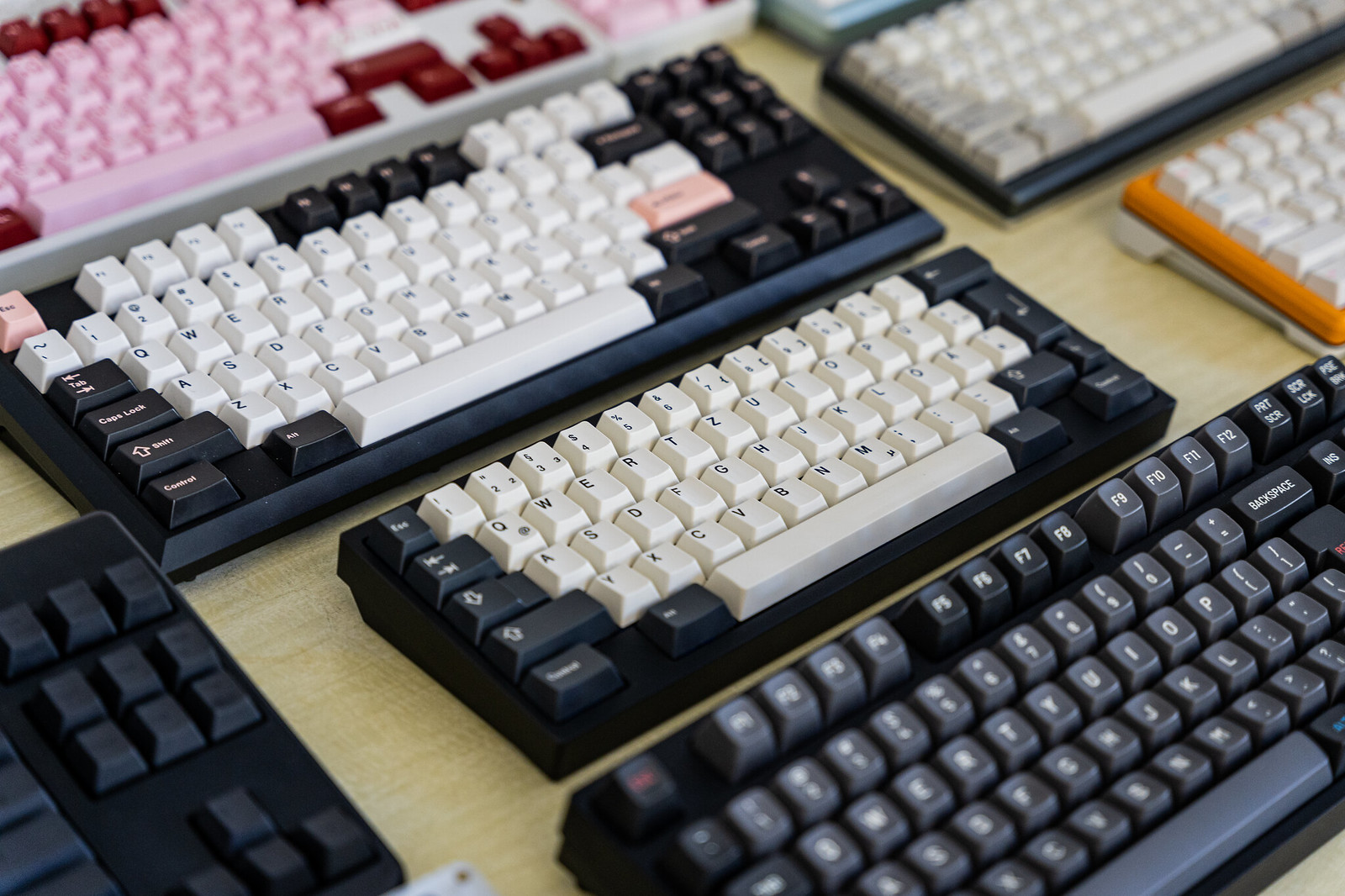The image is a close-up, color photograph of several mechanical keyboards arrayed diagonally across a light-colored table, showcasing a variety of designs and customizations, typically seen at a mechanical keyboard meet. The keyboards are arranged in rows, mostly overlapping, and some are partially cut off by the edges of the photo. Starting from the bottom right, there's a standard keyboard featuring black and gray keys. Moving upwards, there's a compact keyboard with white keycaps and black function keys. Another smaller keyboard, just above, features white keycaps with pink lettering, and black keys for the escape and enter keys. Farther up, a keyboard boasts a unique mix of white keycaps with pink and red keys. In the top left corner of the photo, a keyboard stands out with an entirely white base and pink and dark red keys. On the top right edge, there are hints of additional keyboards, including one with an orange border and white keys, and another with a blue border. Each keyboard presents a distinct combination of keycap colors and layouts, reflecting the diverse customization preferences of mechanical keyboard enthusiasts.